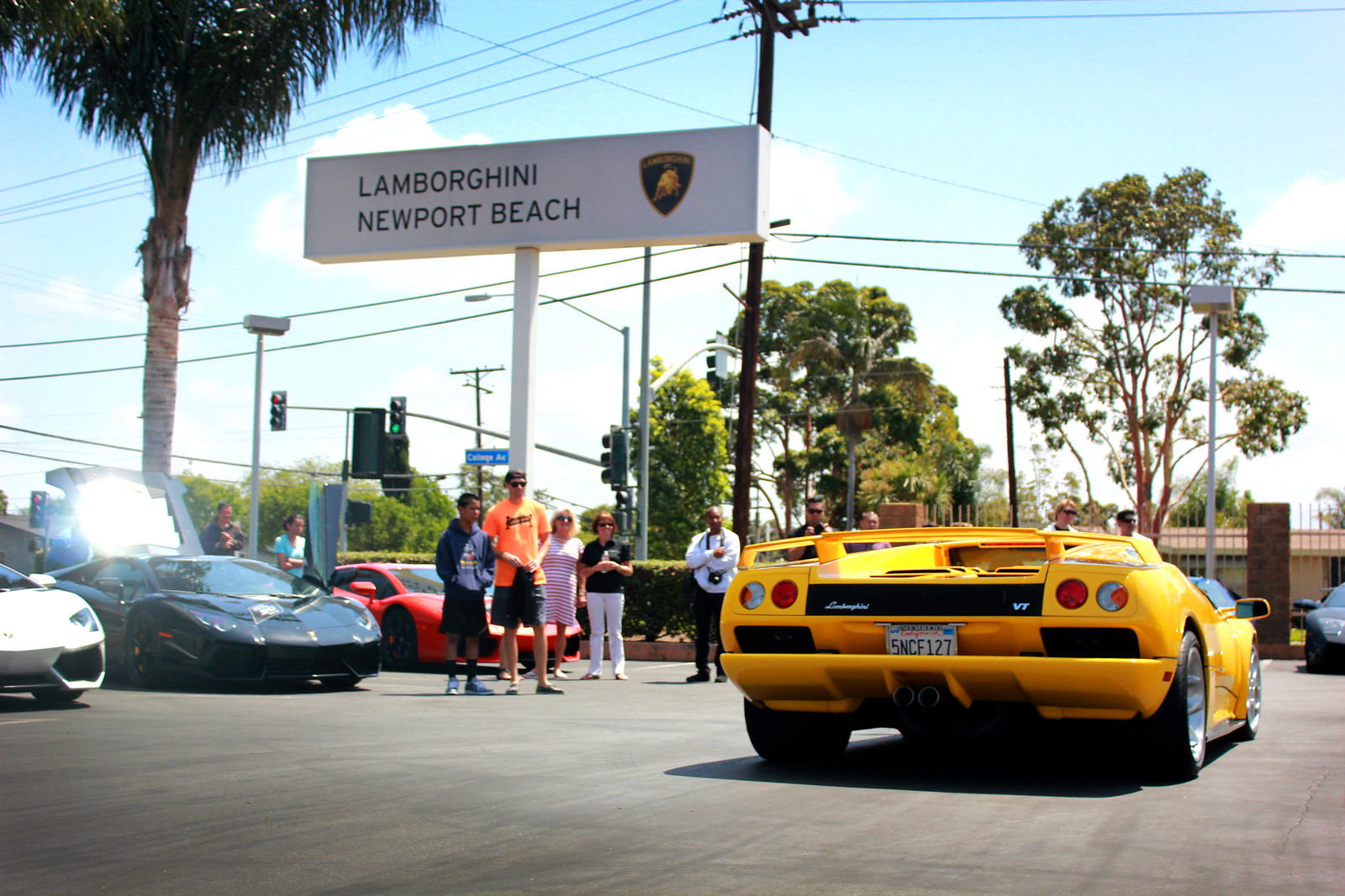On a bright and sunny day with a clear blue sky dotted by a few white clouds, the image captures the bustling scene of a Lamborghini car show at a dealership in Newport Beach, California. The setting features a blacktop parking lot, with a large white sign to the left that reads "Lamborghini Newport Beach" alongside the iconic Lamborghini logo. The lot is framed by sparse green trees and a tall palm tree on the left, enhancing the Southern California vibe. In the foreground, a striking yellow Lamborghini Diablo, viewed from the rear, stands out with its black rear vent area and distinctive tail lights, capped by a yellow spoiler. Groups of enthusiasts gather around this car, marveling at its design. To the left, additional Lamborghinis in white, black, and reddish-orange hues are lined up, contributing to the luxurious atmosphere of the event. In the background, a set of traffic lights and more greenery subtly integrate the dealership setting with its surroundings.